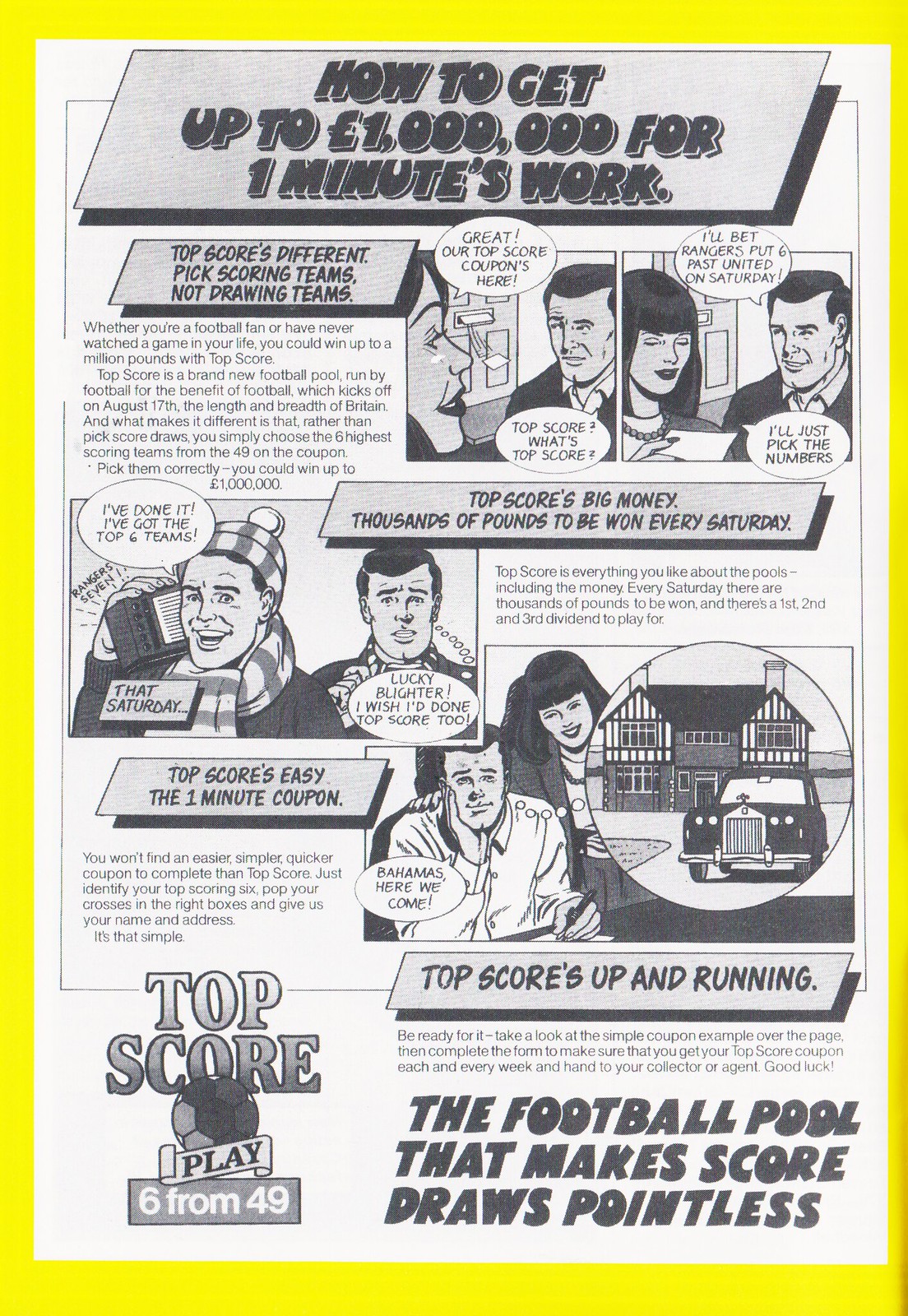This advertisement, designed in a vertical rectangular format, features a prominent yellow border surrounding its content. Within this border lies a comic strip-style layout, rendered in black and white, and split into multiple panels. At the very top of the image, there's an eye-catching parallelogram box with a grayish background and dark lettering that reads, "How to get up to a million pounds for one minute's work."

Beneath this headline, you'll find sequential visual and textual elements organized in a systematic manner. Each section includes cartoon illustrations featuring various scenes with men, women, a car, and a house, accompanied by dialogue and narrative text in smaller print. Directly under the main headline, smaller boxes highlight key points such as:

- "Top scores, different pick scoring teams, not drawing teams."
- "Top scores, big money, thousands of pounds to be won every Saturday."
- "Top scores, easy, the one minute coupon."
- "Top scores, up and running."

The lower part of the image emphasizes the core message of the advertisement with bold text stating, "The football pool that makes score draws pointless." In the bottom left corner, a graphic symbol, likely resembling a soccer ball, bears the phrases "Top score," "Play," and "Six from 49."

This detailed comic strip format combines visual storytelling with enticing offers, effectively promoting the betting business and its lucrative draw system.